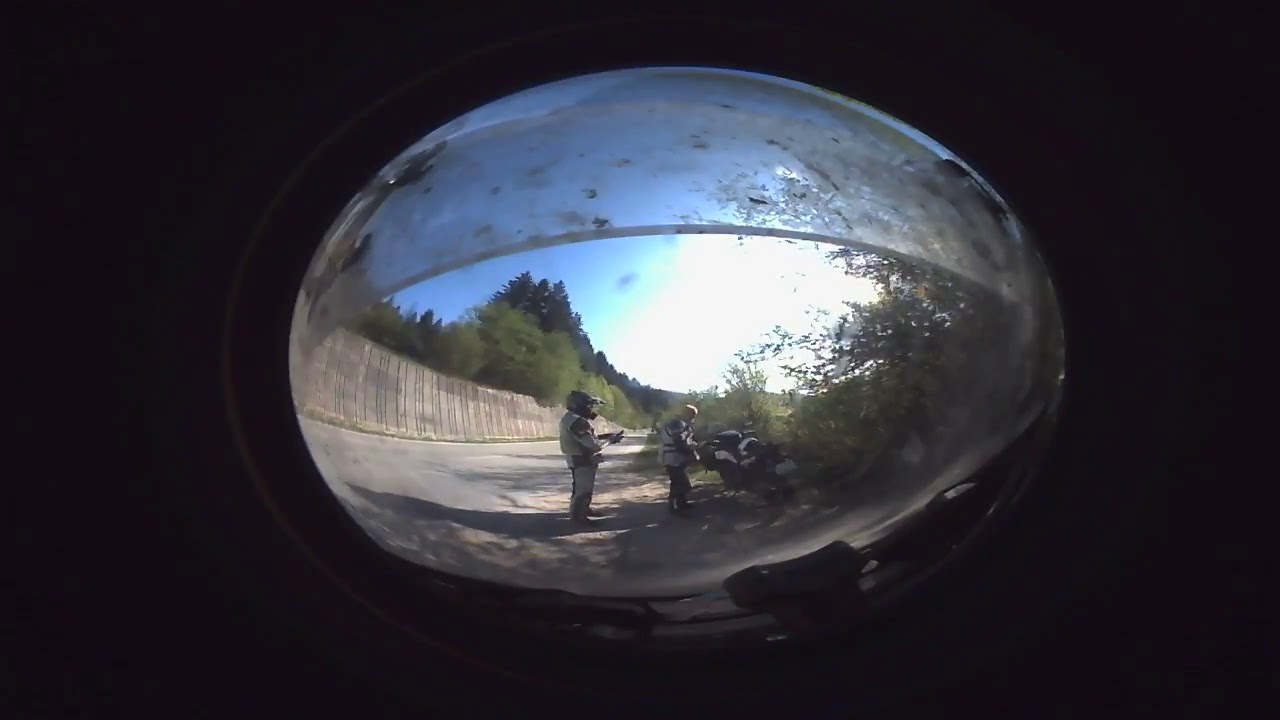The image presents an intriguing scene captured through a distorted, oval lens, evoking the sensation of peering through a small, circular window or possibly the headlamp of a vehicle. The photograph features two people standing beside a motorcycle at the side of a gray road, framed by a tall fence on the left. The person on the left is wearing a black motorcycle helmet, while the person on the right is not. Both are dressed in outfits with dark and gray tones, and the woman on the right dons a puffy gray jacket.

The background reveals a picturesque blend of greenery with trees and bushes, and a sky transitioning from blue on the left to white on the right, suggesting the sun is rising. The image has a peculiar overlay resembling a translucent plastic or wax paper covering, particularly dirty and stained at the top half, adding to the overall mysterious and aged appearance of the scene. The entirety of the image is encased in a black, oval-shaped border, further enhancing its encapsulated and slightly surreal quality.